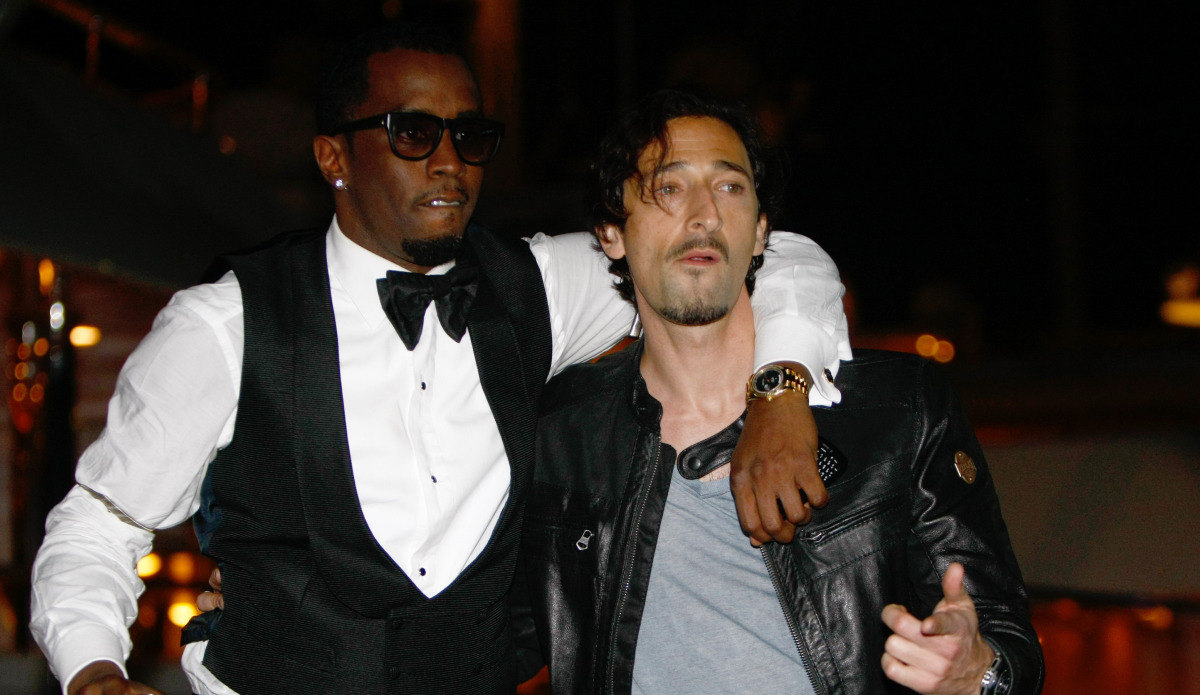The photograph captures two famous male actors posing together outside at night, set against a backdrop illuminated by a warm glow. The actor on the left is a black man with short, edged-up hair, dark facial hair including a goatee, and a white gold stud in his ear. He dons black glasses and a tuxedo-like outfit with a white dress shirt, black bowtie, and a black vest. His arm is draped around the other actor. The man on the right has dark brown, medium-length hair that partially falls over his face, a goatee and mustache, and is wearing a black leather jacket adorned with a gold stud on the arm, over a gray v-neck t-shirt that reveals some chest hair. His hand is playfully pointed out in a gun-like gesture. Both actors are casually looking off to the side, seemingly relaxed and unaware of the camera capturing this candid moment.